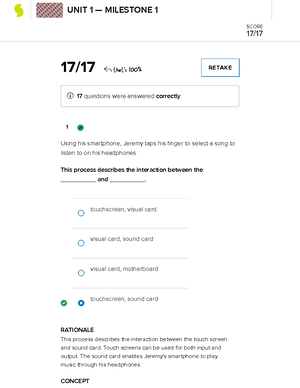Screenshot of Online Quiz Result Page for Unit 1-Milestone 1 with Perfect Score

At the top left corner of the image, a logo features a green 'S' symbol. Adjacent to the logo, the text "Unit 1-Milestone 1" is prominently displayed in bold black, followed by the impressive score of 17 out of 17. Beneath this, smaller text confirms that 17 questions were answered correctly. A blue button labeled "Retake" is available, indicating users have the option to retake the quiz.

The screenshot shows the questions and answers section, where only the first question is visible. The question reads: "Using his smartphone, Jeremy taps his finger to select a song to listen to on his headphones. The process describes the interaction between the blank and the blank."

Four multiple-choice options are provided:
1. Touch screen and visual card
2. Visual card and sound card
3. Visual card and motherboard
4. Touch screen and sound card

The final option, "Touch screen and sound card," is marked with a green check mark, denoting it as the correct answer.

An explanation below the answer elaborates: "The process describes the interaction between the touch screen and sound card. Touch screens can be used for both input and output. The sound card enables Jeremy's smartphone to play music through its headphones."

At the footer of the image, the section is labeled "Concept," suggesting this segment offers further context about the concept tested in the question.